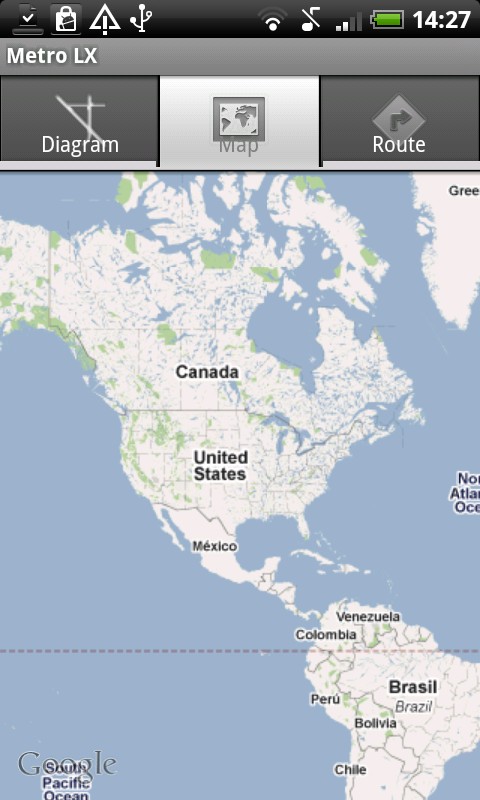This is a highly detailed screenshot of a mobile phone displaying a map application. At the top of the lengthy vertical image, there is a rectangular gray bar spanning the width of the screen, serving as a menu labeled "Metro LX" in white font. Directly below this bar are three square buttons: the first labeled "Diagram," the middle one labeled "Map," and the third labeled "Route." 

The main portion of the image is dominated by a map displaying a broad geographic area that includes North and South America. Key regions and countries visible on the map are Canada, the United States, and Mexico, with the expansive blue of the Atlantic and Pacific Oceans flanking the continents. South America is also prominently featured, with Brazil, Peru, Bolivia, Chile, Venezuela, and Colombia clearly marked. The detailed depiction offers a comprehensive view of this significant portion of the Western Hemisphere.